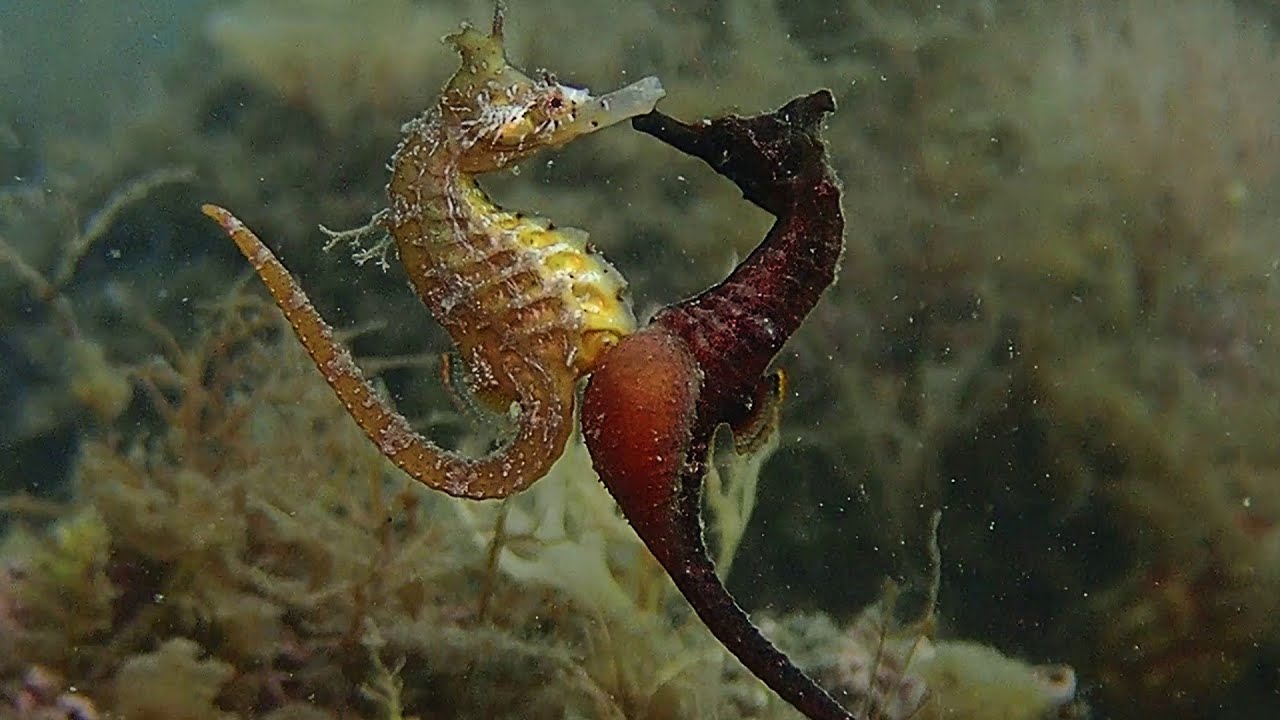In this captivating underwater photograph, two seahorses are seen gently facing each other, their beaks almost touching as if sharing a tender kiss, forming a heart-like shape with their bodies. Set against a backdrop of murky water interspersed with varying hues of seagrass and underwater plants, the scene captures the serene beauty of marine life. The seahorse on the left boasts a yellow body with brown accents, and sits slightly higher in the frame. Its counterpart on the right features a striking dark brown or black body with a lighter brown belly, accented by subtle highlights of red and yellow, adding to its intricate appearance. The blurred background showcases an array of beige and brown plants, creating a natural habitat with minute bubbles that enhance the enchanting atmosphere.